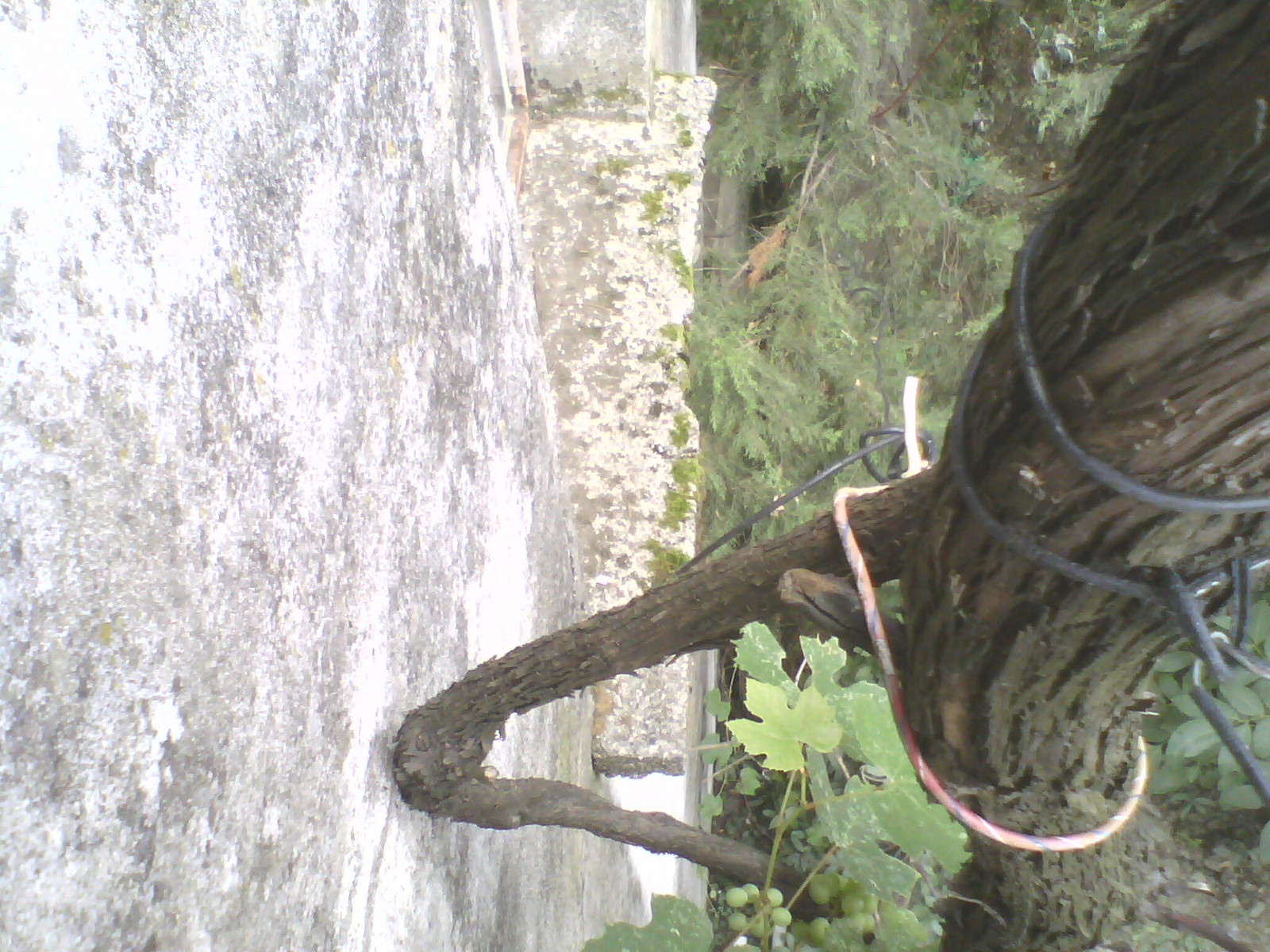This photograph, oriented on its side, captures a detailed scene of a fallen tree resting against a large, aged cement wall, which is gray and white with visible moss or mold at its base. The setting is outdoors in daylight, with sunlight illuminating the image. Prominently, a medium-sized tree trunk appears to be supported by a branch forming a V-shape, which is in contact with the wall. The tree is entwined with both metal wire and multicolored fabric rope, possibly used by specialists attempting to stabilize or remove it. Additional foliage, including fir tree branches, and grapevines with small grapes and grape leaves are visible below the tree. Despite the challenging sideways angle, the image hints at a wooded area beyond, separated by a concrete structure that could resemble an empty pool or a pathway, suggesting a scene following a storm.